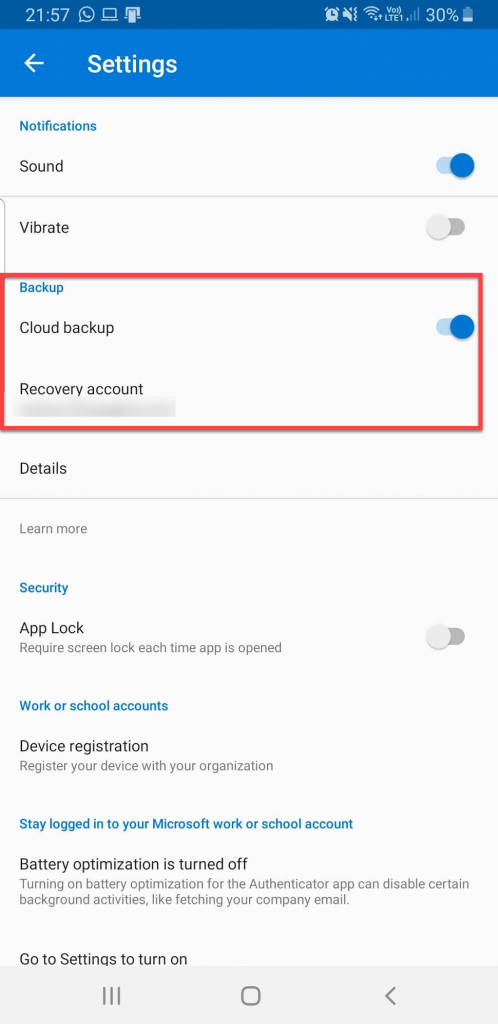A detailed screenshot of a phone's settings menu taken at 21:57 (9:57 PM). The phone is experiencing low LTE signal strength with only one bar and has 30% battery remaining. The Settings page features a blue bar at the top with white text displaying "Settings" and a back button. 

Below that, the screen shows various settings and notifications:
- **Notifications**: Blue button present.
- **Sound**: Displayed in black, the sound is turned off.
- **Vibrate**: Also turned off.

An instructional section highlighted in red shows:
- **Backup**: Enabled, indicated by black text.
- **Cloud backup**: Turned on, shown in black text.
- **Recovery account**: Button located below the backup section.
- **Details**: Black button.
- **Learn more**: Gray text option available.

Further down, the screen highlights security settings:
- **Security**: Blue button present.
- **App lock**: Security feature, requiring screen lock each time it is opened, is turned off.
- **Work or school accounts**: Blue text with options for device registration.
- **Register device with your organization**.
- **Stay logged into your Microsoft work or school account**: Blue text.

The last section concerns battery optimization:
- **Battery optimization**: Currently turned off. A note indicates that enabling this might disable certain background activities, such as fetching company emails.
- **Instructions to enable battery optimization**: Directs the user to go to settings.

At the bottom of the screen are the standard menu, home, and back buttons, typical for most smartphones. This detailed depiction encompasses various functionalities and statuses within the phone's settings menu.